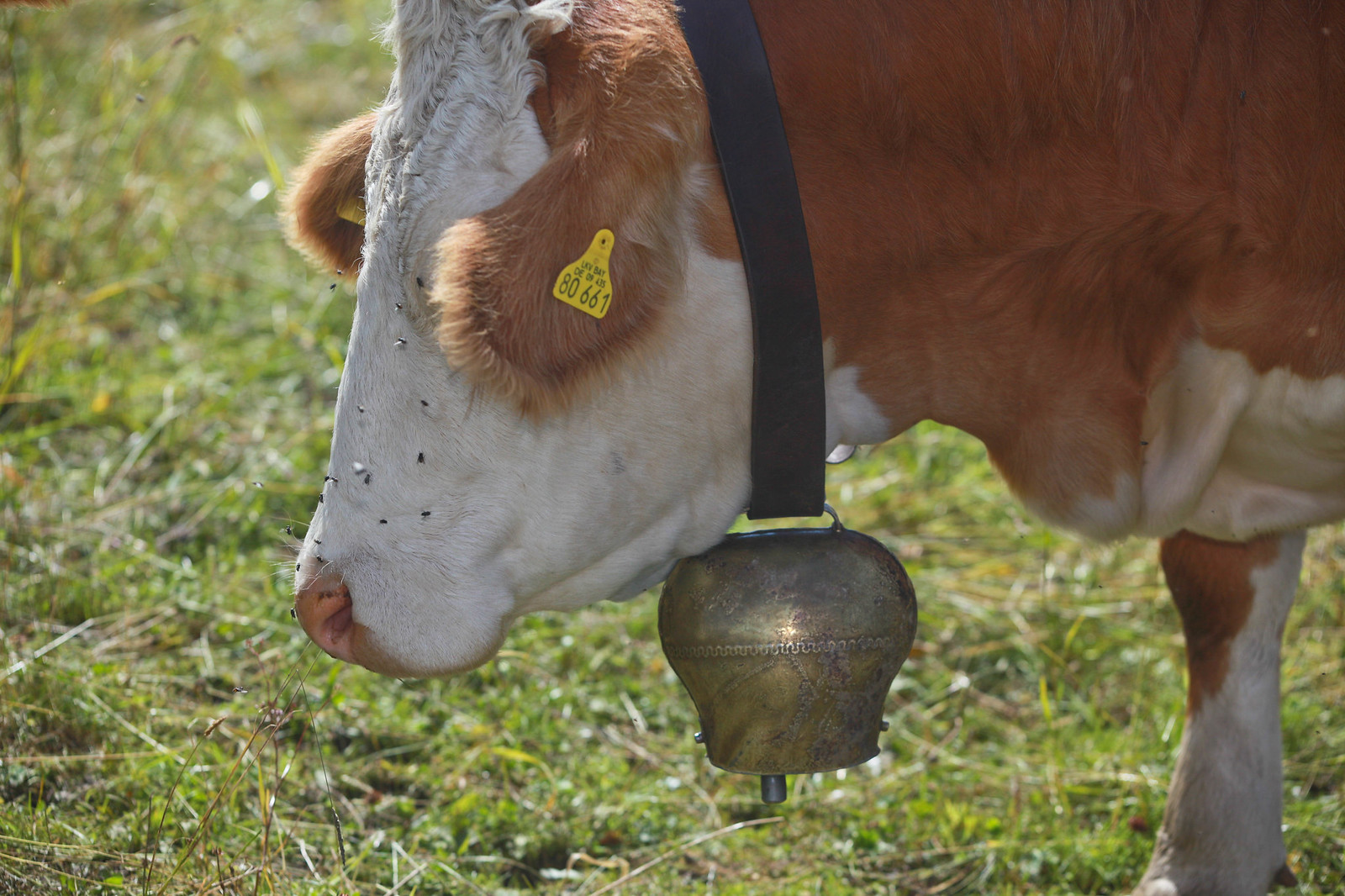The image features a close-up view of a cow, likely a dairy cow, standing still in a grassy meadow. The cow is predominantly white with sable-colored ears and body, and has a pink nose. Its ear is tagged with a yellow ear tag, indicating it is part of a herd. The cow's head is lowered slightly, with its red, fuzzy ears covering its eyes. A notable feature is the large, heavy bell hanging from its neck on a thick black collar, and the bell has a brass or pewter-like appearance with its interior visible. The cow also has excess skin under its neck and chest area. The cow's face and nose are swarmed with small black flies, suggesting a warm day. The grass around the cow appears long and green.